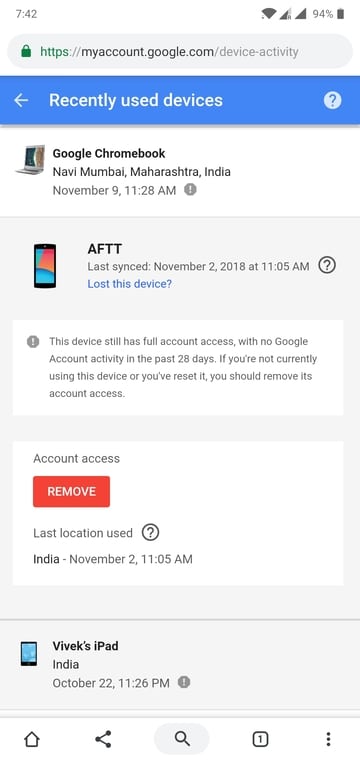A close-up image of an Android mobile phone screen taken at 7:32. The phone is connected to Wi-Fi and is displaying the mobile data symbols for both 4G and 5G connectivity, with the dual SIM indicator visible in the lower right-hand corner. The battery level is at 94%. The phone's screen shows a web browser open to the URL https://myaccount.google.com/.deviceactivity, which details recent device activities associated with a Google account. Visible on the screen are details of a Google Chromebook accessed in Navi Mumbai, Maharashtra, India on November 9th at 11:28 AM, a mobile phone named AFTT last synced on November 2nd, 2018, at 11:05 AM, and an iPad belonging to a user named Vivex with the last activity from India on October 22nd at 11:26 PM. Among the options shown, there is a button reading "Lost this device?" to remove account access if the device is no longer being used.